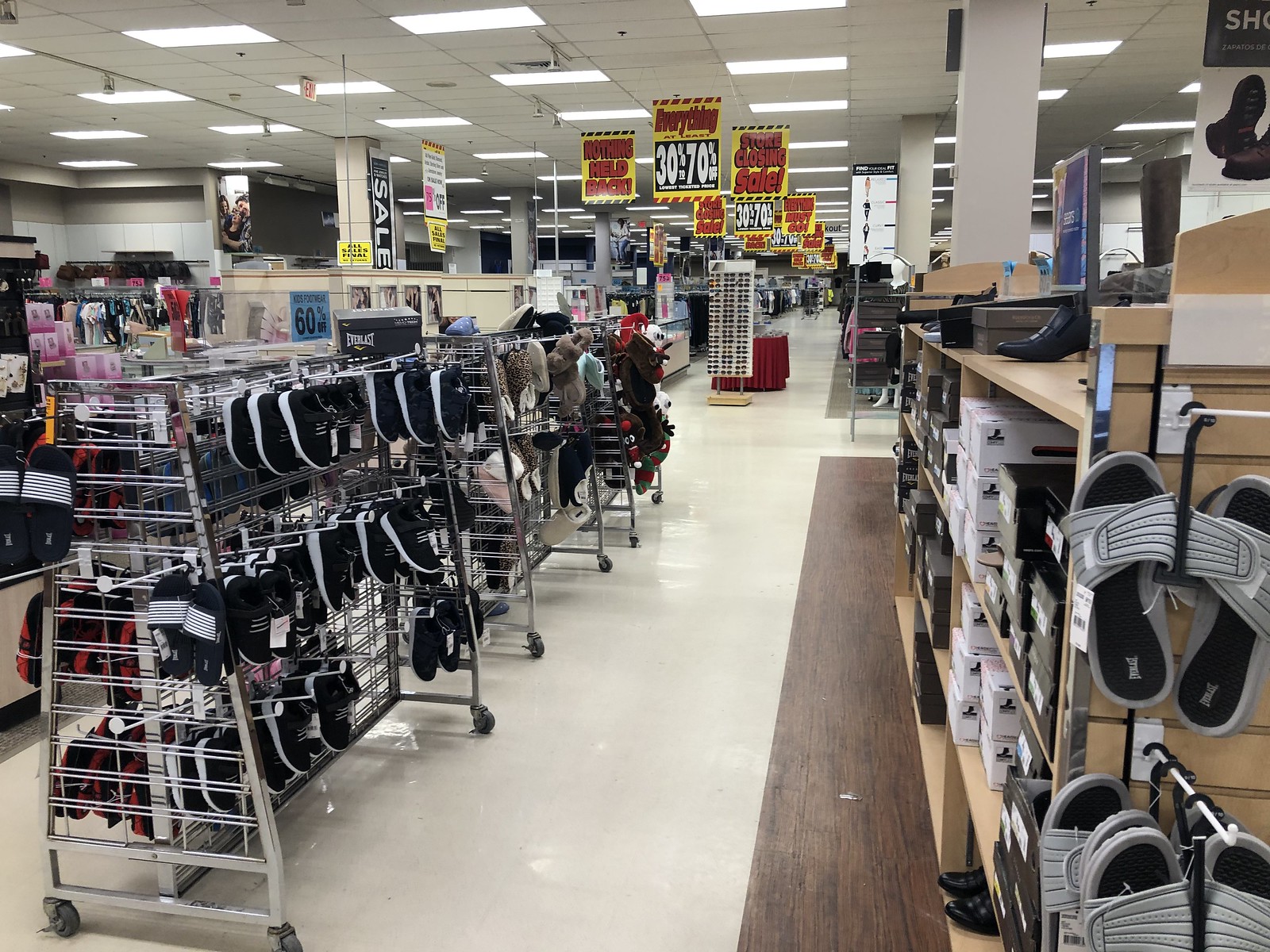In this photograph, we are presented with an interior view of a large box store undergoing a store closing sale. Hanging from the acoustical tile ceiling is a prominent sign reading "Everything 30 to 70% Off, Store Closing Sale." We are situated in the shoe department. On the shelves, there are a variety of footwear options, including a selection of beautiful sandals and some fancier footwear displayed on the top shelf to the right. Simpler sneaker-style shoes with white soles and fabric tops, branded Everlast, are hanging on racks marked at 60% off. Slippers are also visible on a wheeled rack.

Centrally located in the aisle is a display of sunglasses alongside a "Sale" sign. Gazing down the center aisle, we get a clear view of the adjacent clothing department and the electronics department with their display cases. Everywhere, signs declare "Everything must go" due to the store closing. The floor is tiled, and in the distance, a seemingly endless array of items on sale is visible. Banners announcing sales hang throughout, extending the entire length of the store, contributing to the atmosphere of a final, all-encompassing clearance.